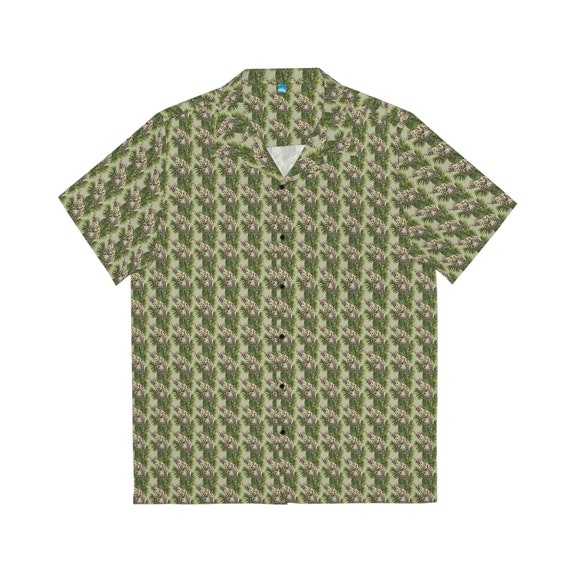In the image, we see a detailed, color illustration of a men's short-sleeved button-down shirt with a standard collar. The shirt is depicted against a stark white background, giving the impression that it is floating, much like a product photo seen on e-commerce websites. The shirt features a distinctive pattern: green striping that resembles shrubbery runs vertically, interspersed with beige flower-like designs. These elements are set against a light sage green background. The shirt, made of a cotton and rayon blend, is designed with small black buttons running down the front and a squared-off bottom hem. Notably, the center of the collar reveals a white triangular shape, possibly tissue paper, enhancing the realism of the illustration.